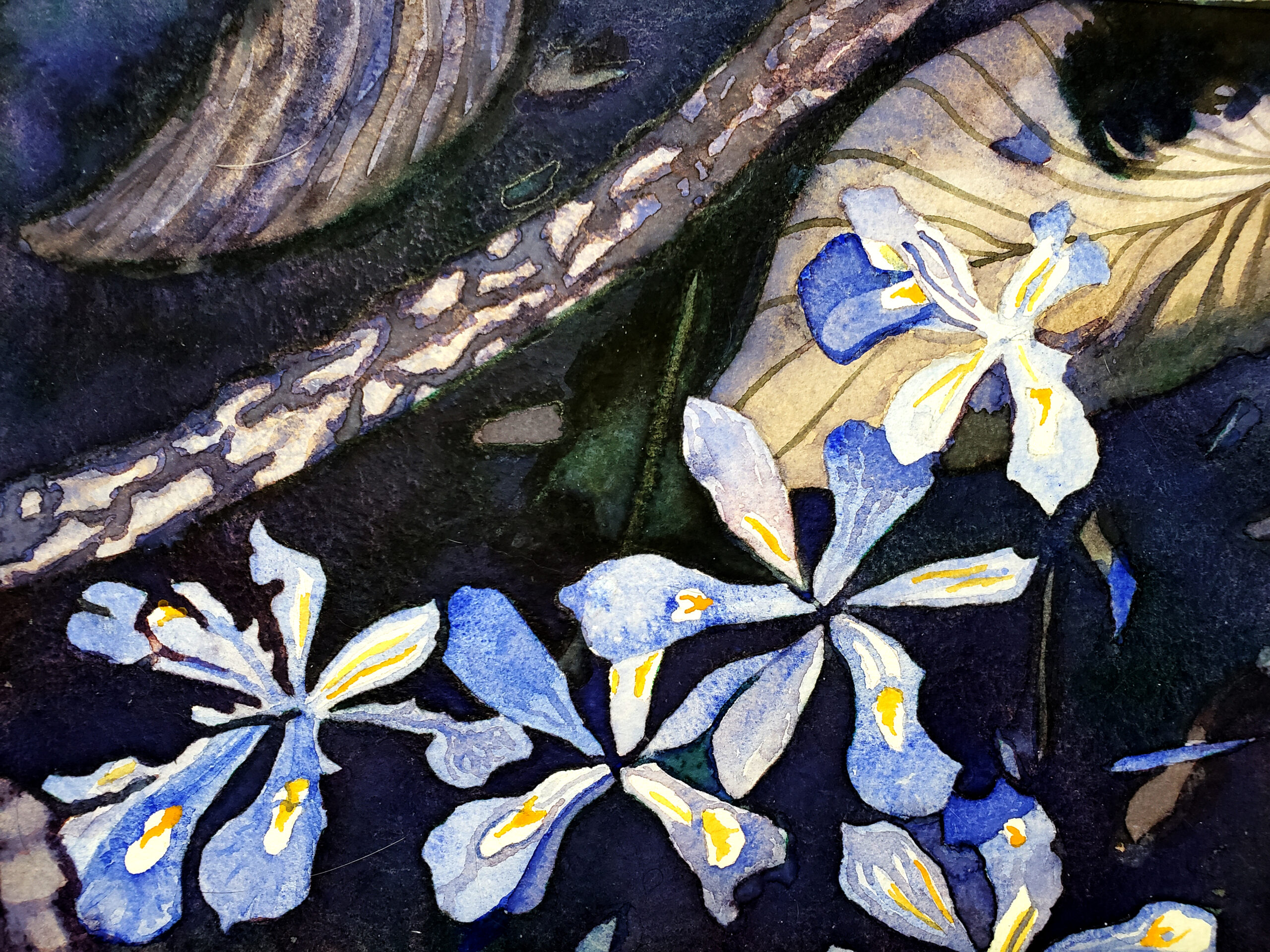This painting of irises features a prominent dark blue and black background, which sets off the vivid details of the composition. Five blue flowers with yellow and white accents on their petals are arranged across the lower right and bottom portions of the canvas. Each flower exhibits gradual transitions of color, drawing the eye to their intricate beauty. In the upper right corner, a large leaf painted in green, yellow, and white curls downward, adding a sense of movement with its striped appearance. To the left of this leaf, a tan and brown branch, resembling a rope, meanders through the composition. Additionally, a snake-like figure marked with white camouflage and possibly a white eye can be spotted near the upper left, enhancing the mysterious aura of the scene. The interplay of colors and textures, from the dark, almost aquatic background with hints of green, to the delicate flowers and dynamic foliage, invites viewers to explore and ponder the layered, possibly symbolic elements of this artwork.